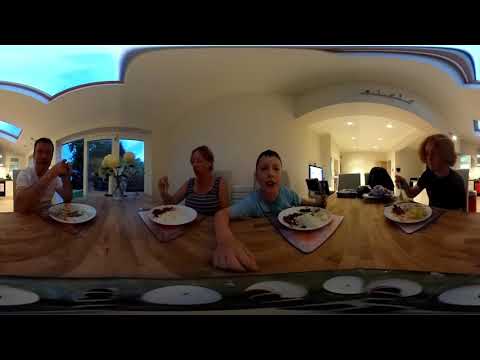In this horizontally rectangular image, a family of four—all Caucasian—are seated at a wooden counter, which appears warped and curved due to the use of a panoramic or 360-degree camera. The counter, composed of light brown rectangular slats, features prominently in the foreground, drawing attention to the white plates piled with food, likely rice and meat. From left to right, there's an older man, a woman, a young boy who is looking directly at the camera, and another young man.

The setting is a white-walled restaurant, as suggested by the white concrete building in the background with large windows on the left side and a curved, flowery top. A TV is noticeable on the right side of the image, indicating a casual dining environment. The ceiling features skylights, allowing the blue evening sky to be visible, hinting that the photograph was taken around dusk. Yellow flowers adorn the table, adding a touch of color to the warm, family-centric scene.